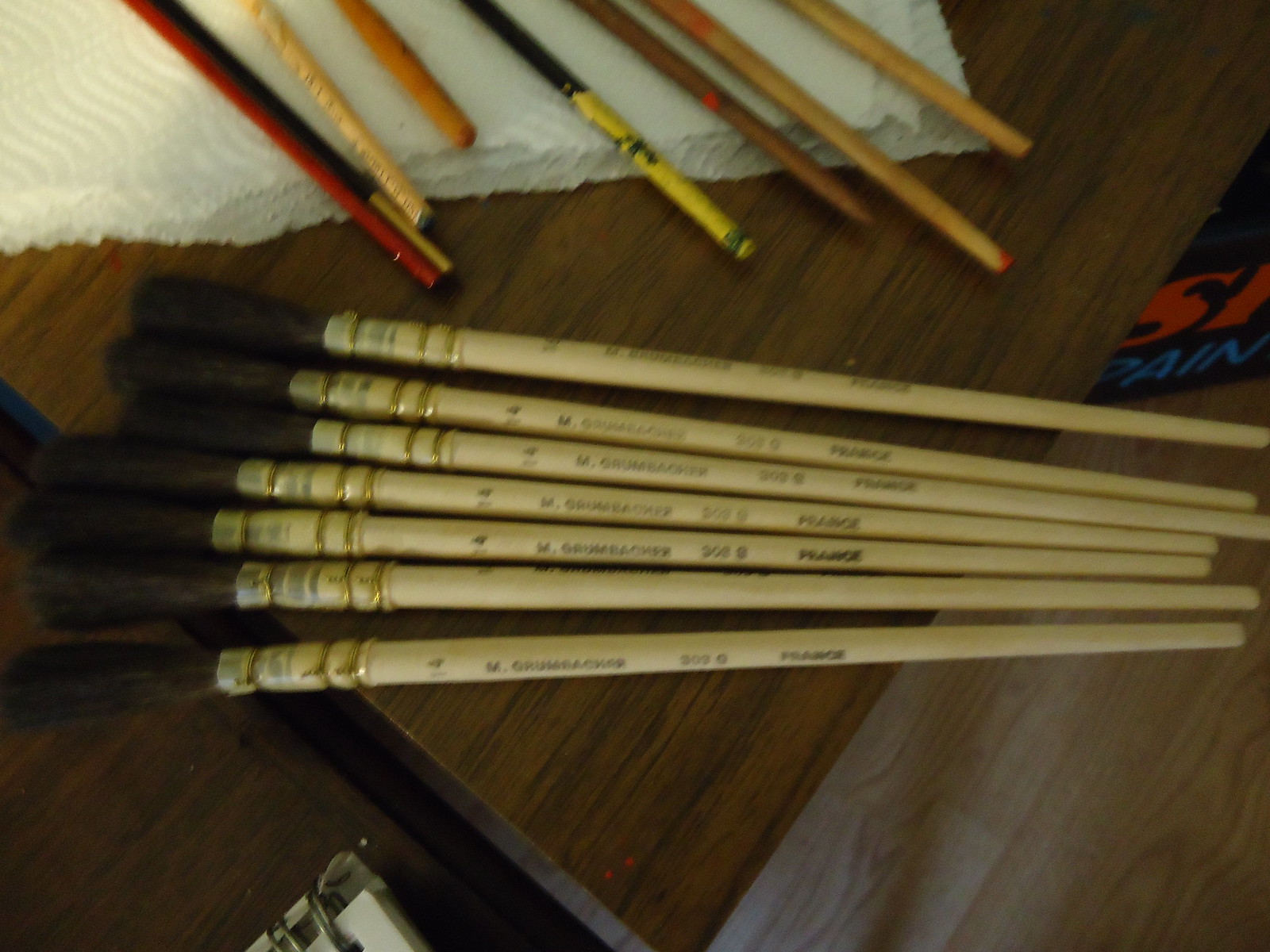The image showcases a dark brown wooden desk seen from an isometric top-down perspective, contrasting with the light brown flooring beneath. At the center of the desk lies a neat arrangement of seven paintbrushes. These paintbrushes, oriented horizontally from left to right, feature dark brown brush tips made of what appears to be horse hair, transitioning into smooth, light brown wooden handles adorned with intricately detailed gold metal ties at the junction. The handles bear small, black text that is difficult to decipher but may include the word "France." Above these paintbrushes, a white paper cloth towel, commonly used in kitchens, adds a touch of texture. This towel hosts an assortment of colored pencils and additional thinner paintbrushes in hues ranging from light yellow to black, red, and orange. The overall photograph, slightly blurry, captures a simple indoor setting and is presented in a square format.